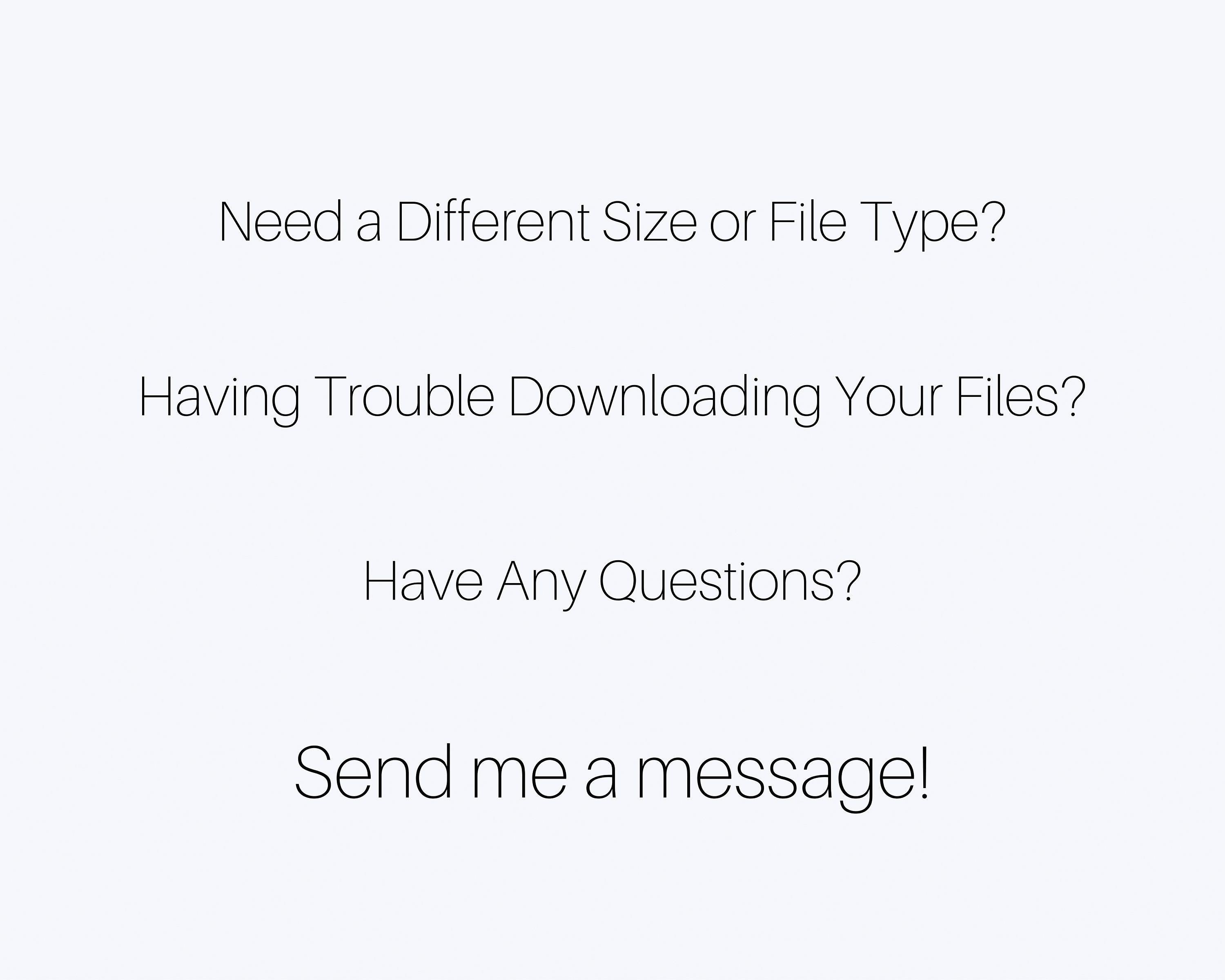This image is a square-shaped screenshot featuring four lines of text against a light gray background, with all text centrally justified, ensuring equal spacing on the left and right sides, as well as consistent space between the messages and the edges.

The text is presented as follows:

1. **"Need a Different Size or File Type?"** - This first line is in title case with black letters, posing a question.
2. **"Having Trouble Downloading Your Files?"** - The second line, also in title case and black letters, follows after a line break, asking another question.
3. **"Have Any Questions?"** - The third line continues the theme in title case and black letters, again ending with a question mark.
4. **"Send me a message!"** - This final line, separated by a space and slightly larger in font size, is in sentence case and ends with an exclamation mark, indicating a call to action.

Each line of text is large and easy to read, designed for clear communication. The image is simple yet effective in conveying its message, with no additional graphics or elements.